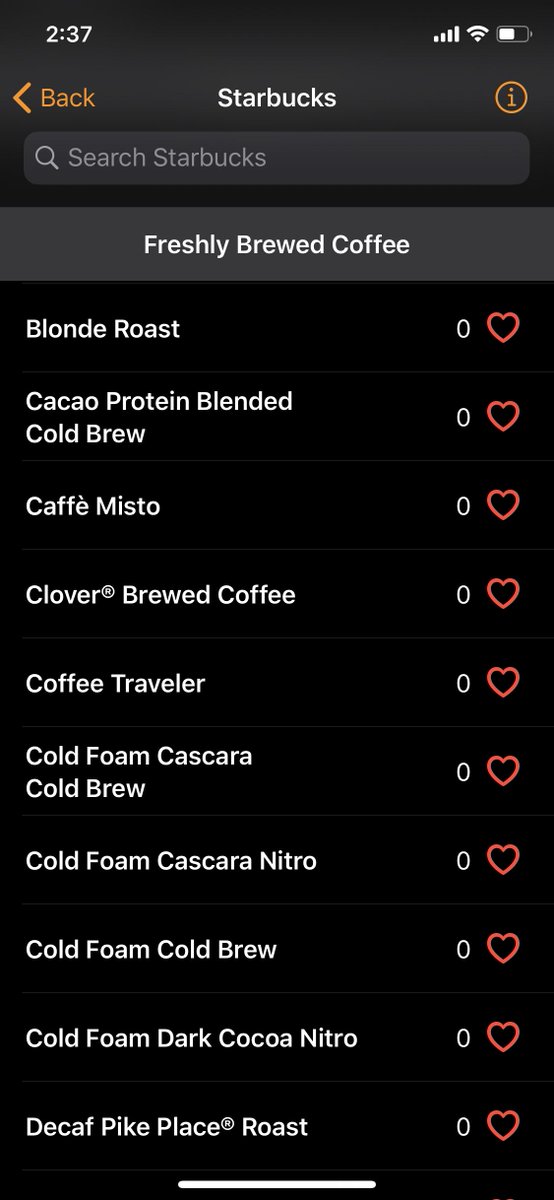This is a detailed screenshot of the Starbucks app displayed on an iPhone with a black iOS background. On the top-left corner, the iPhone time reads 2:37. On the right side of the screen, indicators show four cellular bars, a Wi-Fi connection with three bars, and a battery icon. Below these status indicators is an orange "Back" option, a white "Starbucks" text centered at the top, and an orange information icon represented by an "i" inside a circle.

Directly beneath this top bar is a search bar labeled "Search Starbucks." Following this, there is a menu section. The first item in the menu is a gray box with white text reading "Freshly Brewed Coffee." Below this header, there are 10 menu options, each set against a black background with white text. To the side of each option is an empty heart icon, which users can tap to fill, presumably adding the item to their favorites, changing the count from zero to one.

The 10 options listed from top to bottom are:
1. Blonde Roast
2. Cacao Protein Blended Cold Brew
3. Café Misto
4. Clover Brewed Coffee
5. Coffee Traveler
6. Cold Foam Cascara Cold Brew
7. Cold Foam Cascara Nitro
8. Cold Foam Cold Brew
9. Cold Foam Dark Cocoa Nitro
10. Decaf Pike Place Roast

Each option is separated by a small gray line.